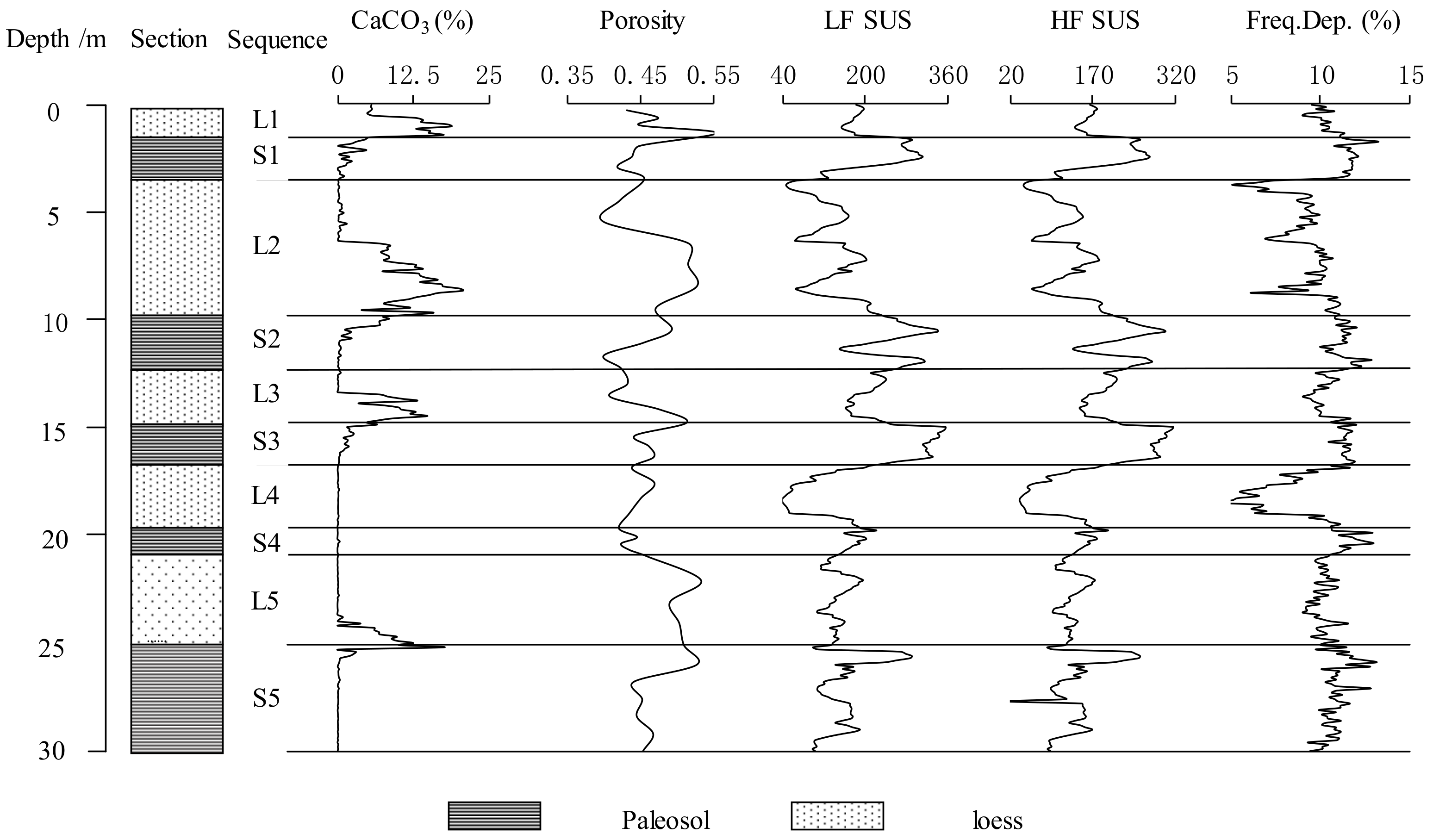This black and white diagram is a detailed mathematical chart illustrating various graphs and measurements. In the top left corner, a scale labeled "depth" ranges from 0 to 30, increasing in increments of five. Below this, the chart is divided into sections and sequences, each with corresponding numerical and categorical data. The sections feature two types of soil, loess and paleosol, represented by different colors and layered patterns. The sequence labels L1, S1, L1, S2, L1, S3, and so forth align with these soil types, with 'L' indicating loess and 'S' indicating paleosol, which is depicted in a darker gray.

The middle and right areas of the chart are populated by various squiggly lines, reminiscent of those from a lie detector graph, which could illustrate attributes such as porosity or chemical contents of the soil. These lines vary in intensity and shape, ranging from jagged and irregular peaks and valleys to smoother curves. Some are darker and more pronounced while others are lighter and less defined. The chart also features several horizontal lines crossing the diagram, adding to its detailed scientific representation of soil properties and sequences.